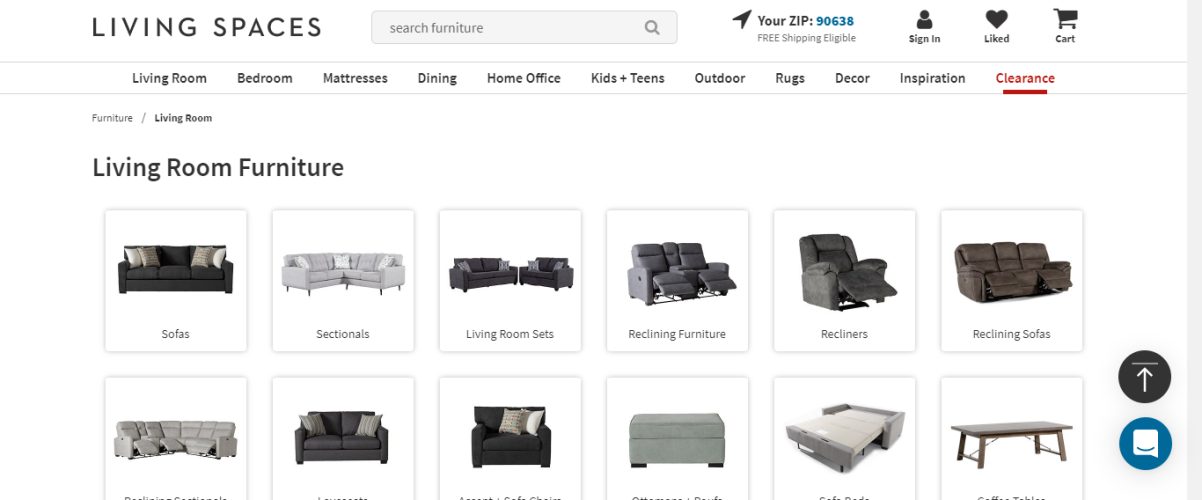The website features a two-tone background, with the left-hand corner in white and the rest predominantly black. Positioned at the top-left corner is the phrase "Living Spaces" displayed in black. Adjacent to this, there's a gray search box with the prompt "search furniture" in lighter gray alongside a gray magnifying glass icon.

Toward the right, a black arrow points rightwards next to the text "Your zip..." in black, followed by "90638" in blue. Below, the phrase "Free Shipping Eligible" is presented in black text.

Lining the top navigation bar from left to right, the following options are listed in black: "Sign In" paired with a silhouette icon, "Like" aligned with a heart icon, and "Cart" next to a shopping cart icon. Underneath these, there is a thin gray line that extends across the page.

Beneath the gray line, the main categories are listed: "Living Room," "Bedroom," "Mattress," "Dining," "Home Office," "Kids and Teens," "Outdoor," "Rugs," "Decor," and "Inspiration," with "Clearance" highlighted in red and underlined, indicating the user is currently browsing the clearance section.

Another thin gray line separates these from the browsing path, which reads "Furniture / Living Room / Living Room Furniture" in black.

The page displays a series of gray-outlined white boxes categorized under various headings: "Sofas," "Sectionals," "Living Room Sets," "Recliner Furniture," and "Recliners." 

The visible products include:
- A gray sectional sofa
- Two grayish-black sofas
- A green ottoman
- A gray pull-out couch
- A brown desk

The bottom portion of the image cuts off, so additional items listed below these aren't visible.